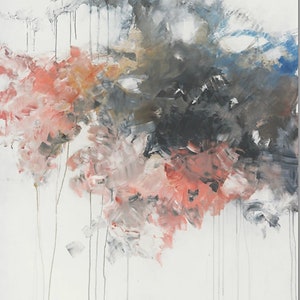This abstract painting features an impressionistic, modern style on a white canvas. Dominated by a blend of colors such as pink, red, black, blue, and gray, the piece presents an intriguing array of droplets and drips cascading down the surface, creating a rain-soaked effect. The composition starts with smaller clusters of flowers arranged in a triangular form at the top left, which gradually grow larger and more prominent as they descend. On the right edge, varying shades of blue and gray enhance the visual dynamic. The bottom portion of the canvas remains predominantly white, with the paint streaks lending an impression of water trickling down, evoking a sense of "rainy flowers on a rainy day." Despite its simplicity, the artwork invites viewers to interpret its abstract forms and color splashes in their own unique ways.